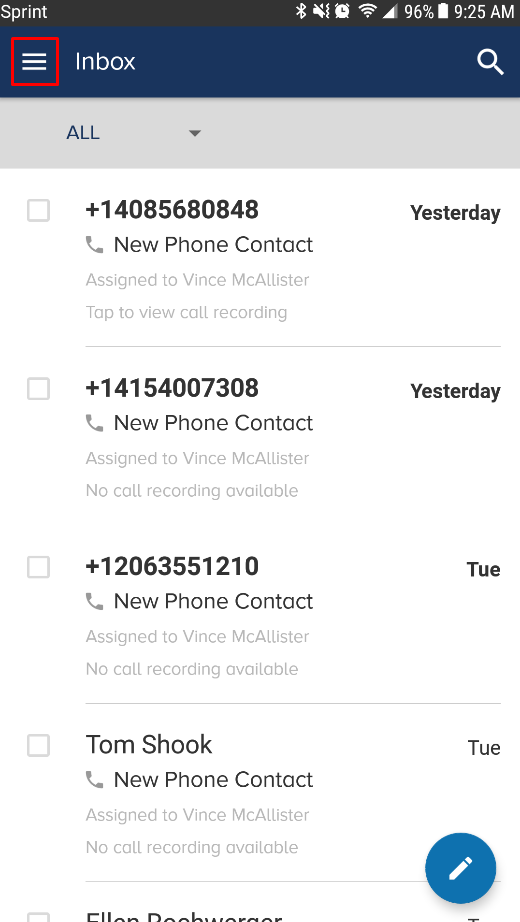The image illustrates the screen of a smartphone showcasing an email or messaging app interface. At the very top, a gray status bar displays essential information, including the carrier name "Sprint," along with various symbols for Wi-Fi, battery percentage, the current time, and Bluetooth connectivity.

Beneath this, the interface transitions into a vibrant blue section labeled "Inbox." Within this area, there's a white magnifying glass icon symbolizing search functionality and a white icon with three horizontal lines, bordered by a red box, likely indicative of a menu or settings option.

The next segment is a gray bar featuring the word "All" accompanied by a small drop-down arrow, suggesting a filter or sorting option for the messages listed below.

The main content area is a white background displaying a list of different messages. Each message is contained within a neat frame with checkboxes, detailing the following:

1. **First Message:**
   - **Phone Number:** +1 (408) 568-0848
   - **Date:** Yesterday
   - **Description:** New phone contact assigned to Vince McAllister. Tap to view call recording.

2. **Second Message:**
   - **Phone Number:** +1 (415) 400-7308
   - **Date:** Yesterday
   - **Description:** New phone contact assigned to Vince McAllister. No call recording available.

3. **Third Message:**
   - **Phone Number:** +1 (206) 355-1210
   - **Date:** Tuesday
   - **Description:** New phone contact assigned to Vince McAllister. No call recording available.

4. **Fourth Message:**
   - **Sender:** Tom Shook
   - **Date:** Tuesday
   - **Description:** New phone contact assigned to Vince McAllister. No call recording available.

In the bottom-right corner of the screen, there's a conspicuous blue circle with a white pencil icon inside, signifying a button likely used for composing a new message or contact.

Overall, the interface is styled with consistent grayscale and blue coloring, providing a crisp layout enhanced by precise black text and user-interactive checkboxes, ensuring functional clarity and ease of use.